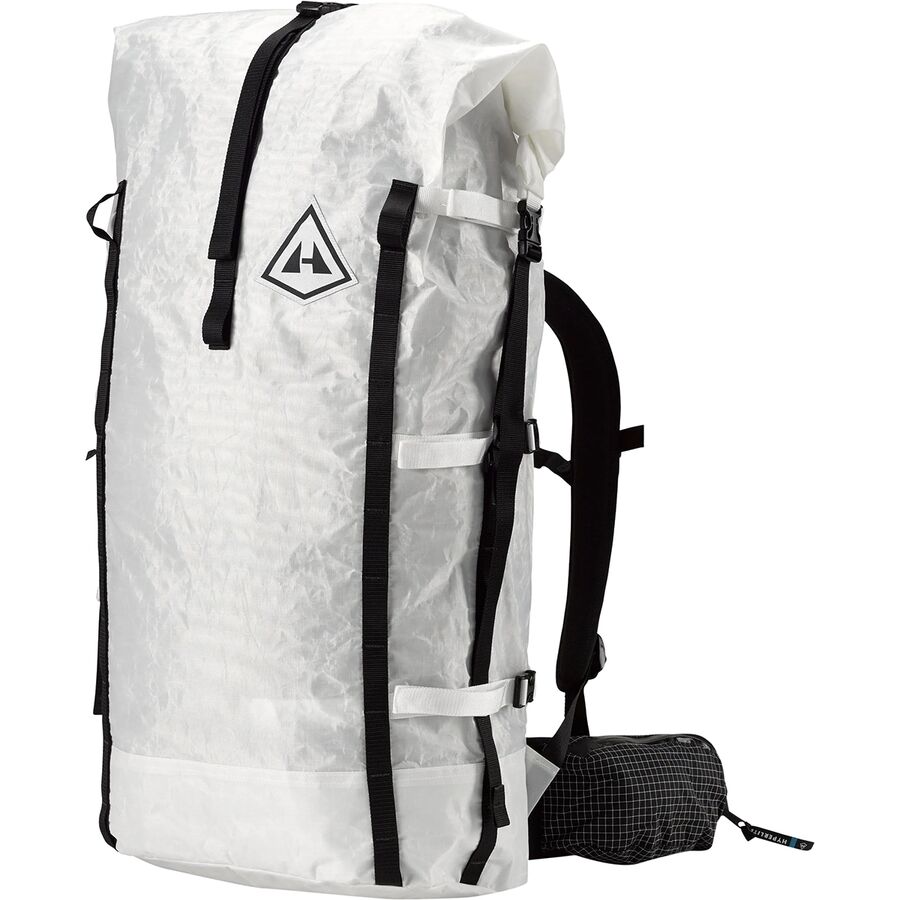The image features a large, heavy-duty, white camping or hiking backpack standing upright against a white background. The bag is rectangular in shape, approximately 3 feet long and 1.5 feet wide. It prominently displays a black triangular logo with an "H" in the middle on the front. The backpack is equipped with multiple black and white straps designed for attaching additional gear and optimizing storage space. The shoulder straps are black and feature a small, attached pouch for extra storage. Behind the main backpack, there is a rolled-up item with a black zipper that appears to be an additional bag or compact accessory.